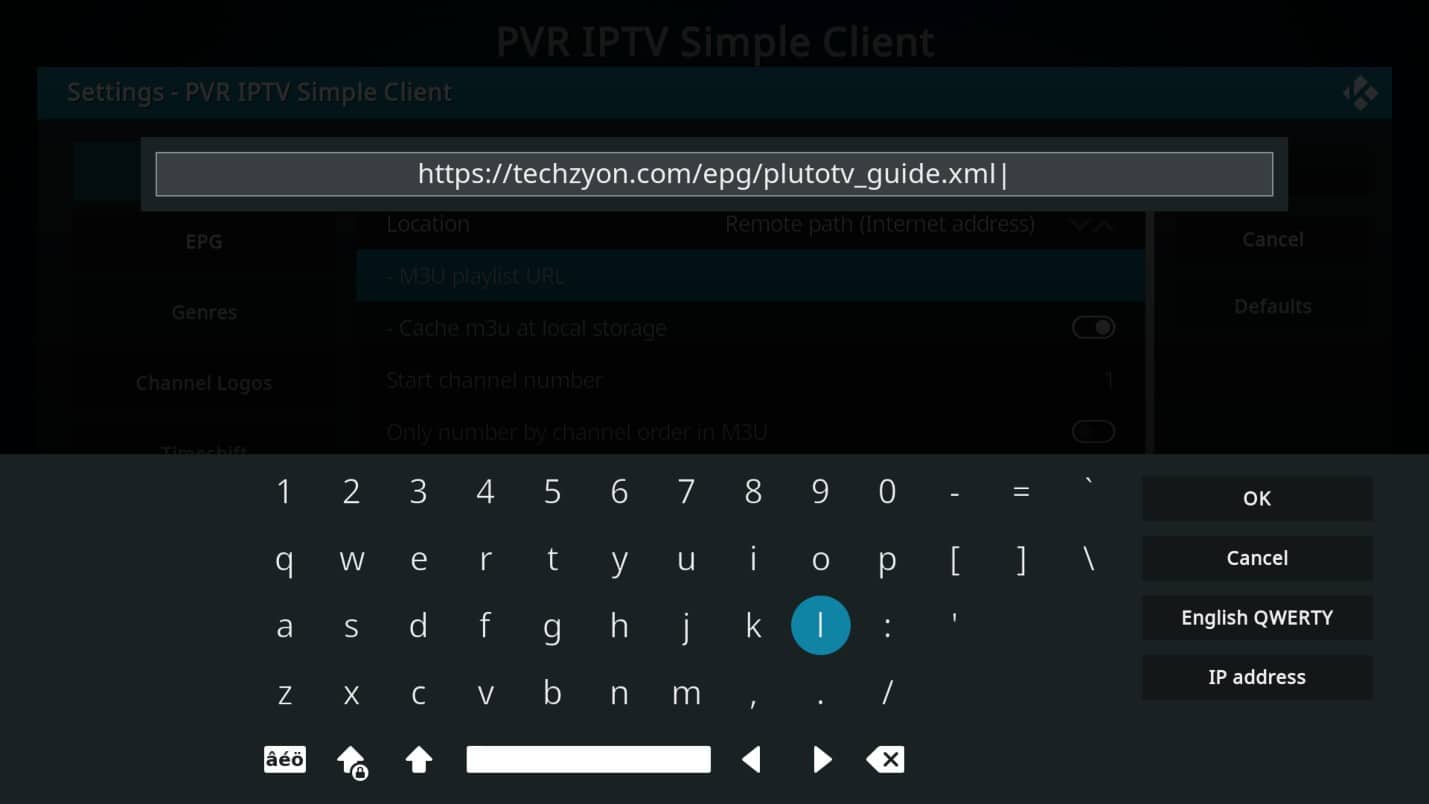In this image, a user is interacting with a website search feature on a dimly-lit screen. The search box is prominently highlighted, making it the focal point of the image. In the background, although obscured by the dim lighting, a settings page is faintly visible, specifically noting "Settings-PVR IPTV Simple Client." The URL entered in the search box is "https://techzion.com/EPG/PlutoTV_guide.xml," and the cursor is positioned at the end of this URL.

Below the search box, an on-screen keyboard is displayed. The letter 'L' is highlighted, likely indicating the next character to be typed. The keyboard layout includes letters, numbers, and symbols such as parentheses, with additional functional keys at the bottom for navigating text input: front and back arrows, the delete key, space bar, and shift key for toggling between lowercase and uppercase.

To the right side of the keyboard, there are four vertically-aligned buttons labeled "OK," "Cancel," "English QWERTY," and "IP Address," providing various options for user commands and keyboard settings. The scene captures a precise moment of user interaction, suggesting the user is configuring settings related to IPTV and inputting a URL for an electronic program guide.